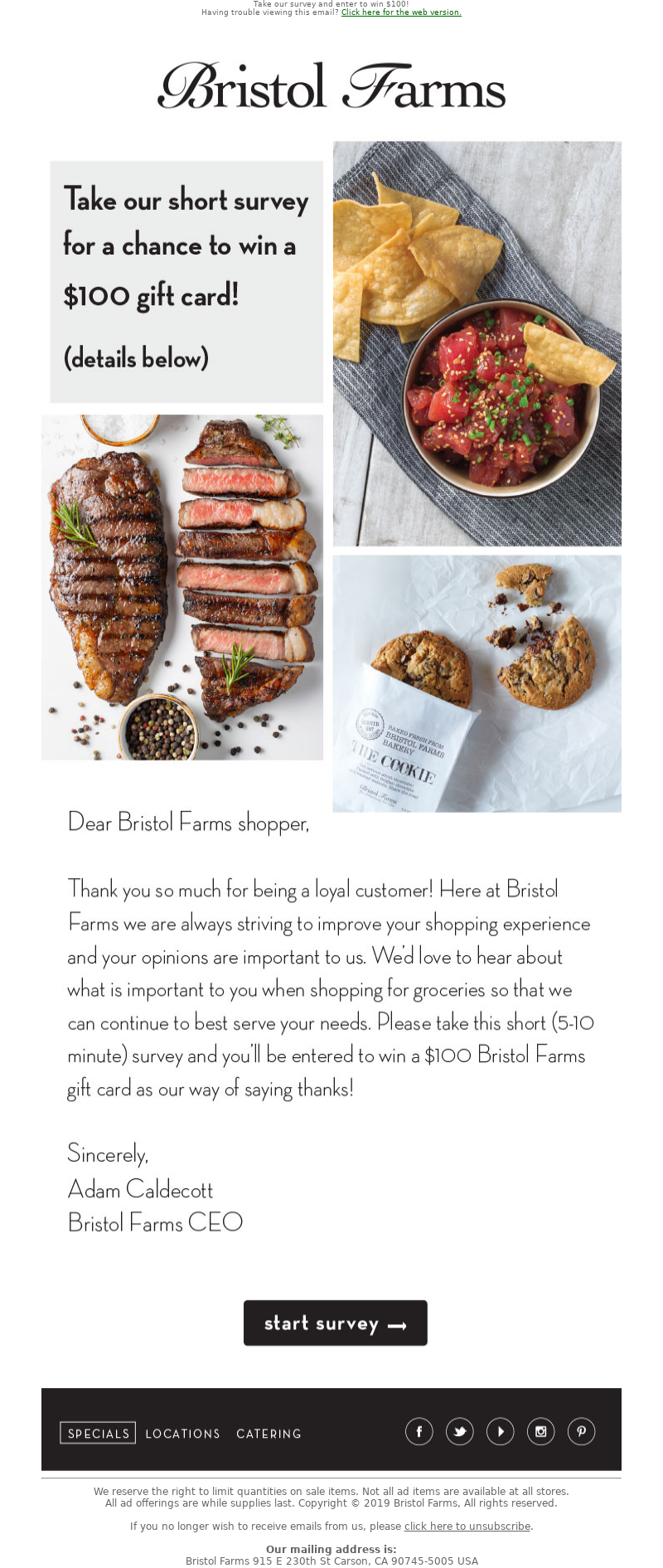**Screenshot of Bristol Farms Website:**

The screenshot captures the homepage of the Bristol Farms website. At the very top, the website prominently displays the name "Bristol Farms." Below this header, there are several images arranged in a grid-like format.

On the top left, there is a banner encouraging visitors to "Take a survey for a chance to win a $100 gift card," with the text "(Details below)" indicating further information is provided elsewhere on the page.

To the right of this banner, an appetizing image of chips accompanied by a bowl of red salsa garnished with green herbs can be seen. The items are laid out on a gray tablecloth.

In the bottom left corner, a visually compelling picture features a piece of grilled meat. The uncut meat on the left boasts deep brown hues with distinct black grill marks and is garnished with fresh herbs. Next to it, on the right, is an image of the same meat sliced open, revealing a succulent, ruby-red interior, showcasing its perfectly cooked state.

In the bottom right corner, there's a close-up of a cookie set, with one cookie nestled snugly in a parchment-like cookie sleeve. Beside it, in the top right section of this image, another cookie is visually broken apart, showcasing its soft and chewy texture with a few bites taken out of it.

Beneath these images, a brief paragraph addressed to the Bristol Farms Shopper starts with a warm greeting and ends with "Sincerely, Adam Cattlecock, the CEO of Bristol Farms," showing a personal touch from the company's leadership.